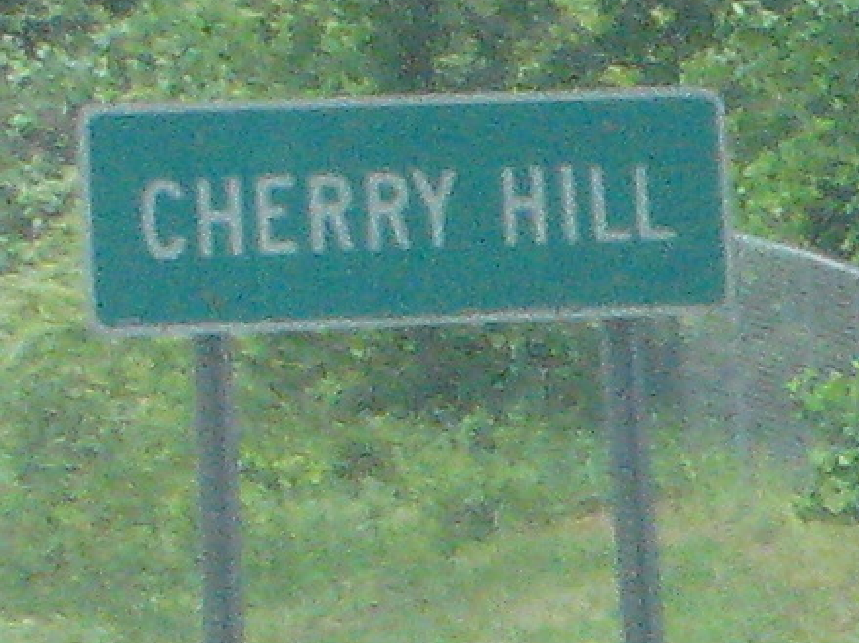In the center of the image, there's a slightly pixelated green rectangular box with a white border, containing white text that reads "Cherry Hill." Flanking the box on either side are vertical steel tubes. In the background, to the back right, there's a visible fence. The entire scene features trees in the background, adding a natural touch to the setting. The overall composition centers around a sign indicating "Cherry Hill."